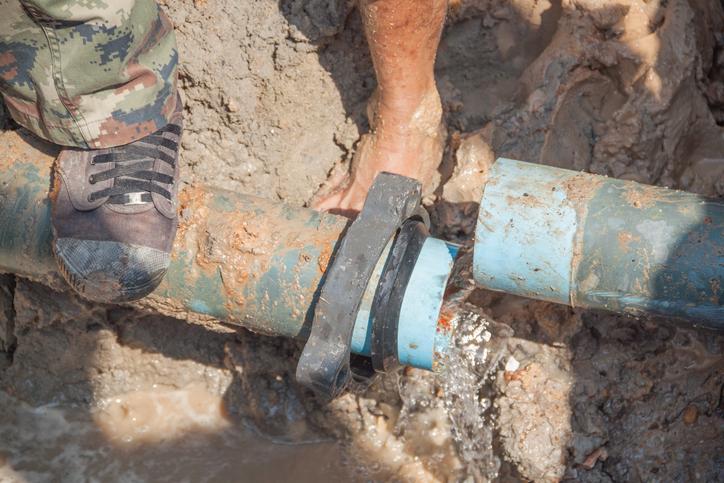The photograph captures a chaotic construction site scene dominated by a muddied, split blue pipe. The pipe spans horizontally through the center, split in the middle, with a section slightly elevated compared to the other. Muddy water drips from the left half of the pipe, saturating the soil with brown, soupy mud. The pipe itself is caked with dirt, featuring varying shades of blue, from a lighter blue at the connection points to darker hues on the outer sections.

In the foreground, a man stands with one foot positioned atop the pipe. His footwear includes what appears to be a heavy-duty sneaker or black Converse shoe, and he is dressed in digital camouflage pants. To the right, another leg, barefoot and covered in mud up to the calf, sinks into the wet soil, adding to the scene's chaotic feel. The overall setting suggests an urgent attempt to manipulate and realign the pipe amid the muddy, waterlogged conditions.